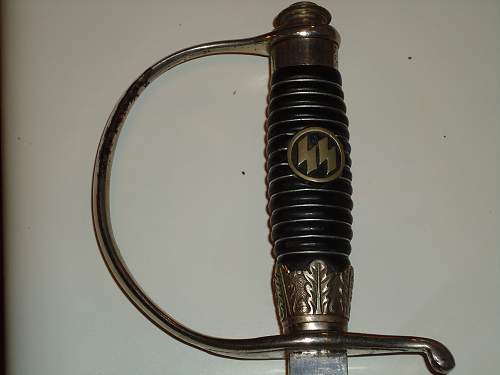The photograph vividly captures a close-up of a sword handle with the blade extending just beyond the frame, pointing downward. The handle, which measures approximately four to five inches in length, features a grip of ridged, dark-colored metal adorned with a metallic leaf flourish near the blade. To the left, there's a prominent, long, arching handguard designed like a half-ring, offering protection to the wielder’s hand. The top end of the handle, where it meets the blade, boasts intricate adornments.

A notable emblem embellishes the grip – two thick, black lightning bolts positioned side by side within a golden circle, an insignia often associated with the SS of Nazi Germany. The overall color scheme of the handle is a blend of dark tones and golden hues, with the metal parts appearing to be either brass or gold. The sword handle is placed against a plain white background, possibly the surface of a table, which starkly contrasts with the detailed and ornate craftsmanship of the handle itself.